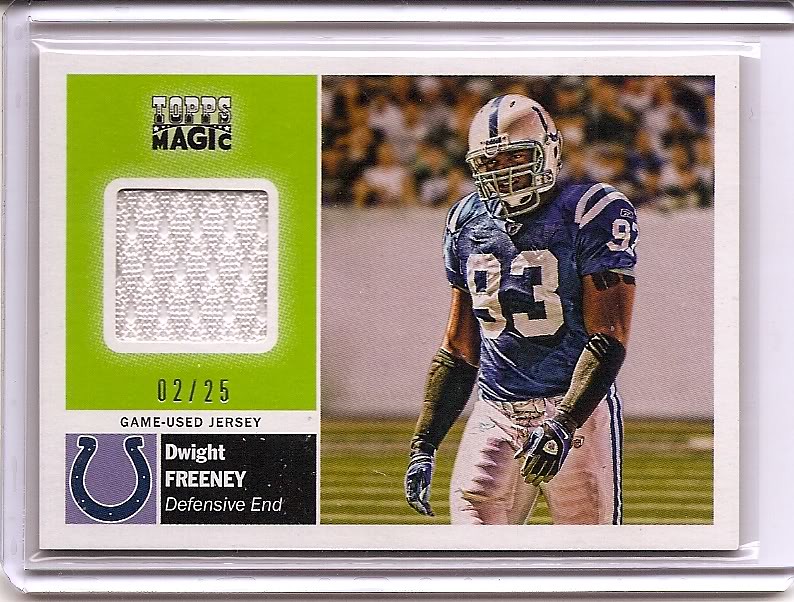The image features a detailed plaque or card encased in clear plastic with white frame borders, likely intended for display. The left side of the plaque has a prominent green, diamond-sparkly area with a square that reads "Topps Magic" in black and white letters. Beneath this square, there is a notation "02/25" indicating the card's limited edition status, along with the words "Game Used Jersey." Additionally, a blue and purple horseshoe logo is present, denoting the player's team. Below this, the name "Dwight Freeney, Defensive End" is displayed inside a dark blue box. The right side of the plaque features an image of Dwight Freeney in his football uniform, which includes a silverish blue helmet, a blue jersey emblazoned with the number 93, white football pants, and black gloves. The photograph captures him on a green field with a blurry background of spectators. The plaque or card appears to be mounted on a white wall, adding to its presentation quality.